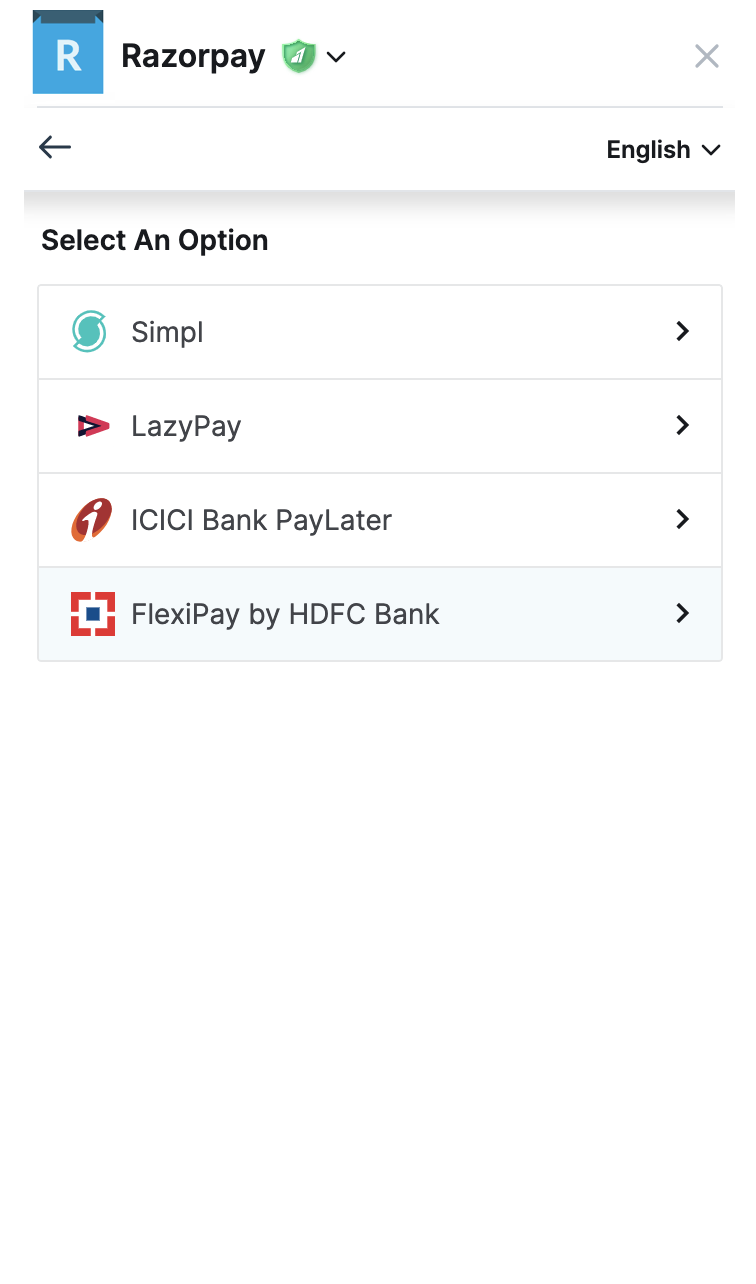The image showcases the Razorpay interface. At the very top, the Razorpay logo features the word "Razorpay" next to a blue box containing a white 'R.' To the right of the logo, there is a small green shield icon. On the far right, there is an "X" button within a downward dropdown menu. Immediately below this, an interface bar includes a leftward arrow on the left side and the word "English" on the far right, paired with a downward arrow indicating a language selection menu.

Further down, there is a section titled "Select an Option" with several payment methods listed in a vertical line. Each option has a rightward arrow indicating further navigation. The options include:

1. Simpl (S-I-M-P-L).
2. LazyPay.
3. ICICI Bank Pay Later.
4. FlexiPay by HDFC Bank.

All text on the page is in black font, while the primary background is white. The page features various colors: blue, two shades of green, red, orange, gray, and black. Notably, the section for FlexiPay by HDFC Bank has a very light blue background, distinguishing it from the others, which are predominantly white.